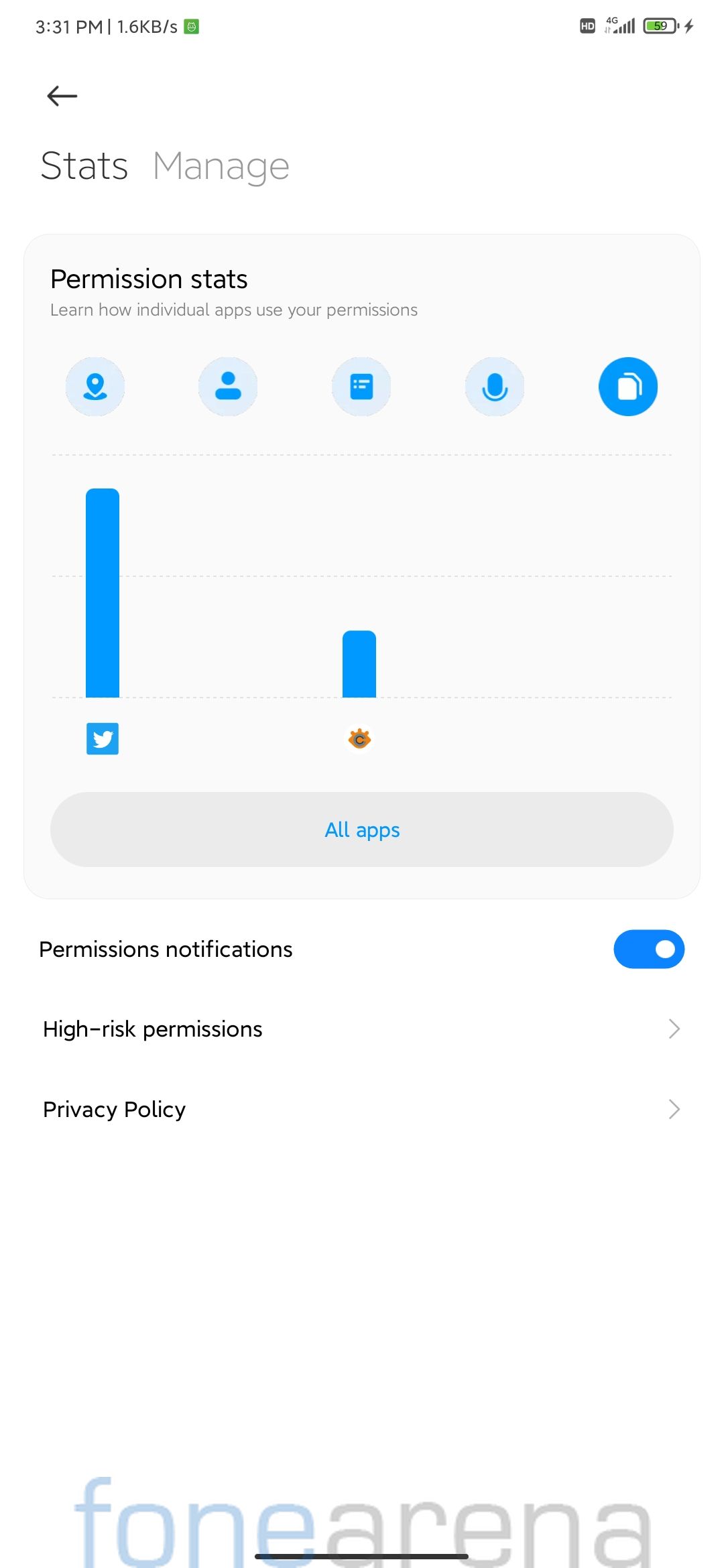Screenshot of a smartphone screen displaying a detailed overview of app permissions and settings. In the top right corner, the status bar indicates a battery icon, an electric symbol, a 4G signal icon, and HD connectivity. The time shows 3:31 PM, with a data transfer rate of 1.6 kb/s.

Below, a navigation panel includes a back arrow, a heading titled "Stats," and a "Manage" option. The main section is labeled "Permission Stats" with the text, "Learn how individual apps use your permissions." Various icons are displayed below: a location marker, a profile image, a text document, a microphone, and a clipboard.

Further down, there's a Twitter icon with a bar above it, followed by a copyright symbol (©) with a smaller bar above it. The section labeled "All Apps" indicates that permission notifications are turned on. Additional options include "High-Risk Permissions" and "Privacy Policy," each with an accompanying arrow for further navigation. The bottom of the screen features the branding "Phone Arena," spelled "f-o-n-e."

This screen provides comprehensive insight into app permissions, allowing users to manage and understand how their information is being accessed and utilized by individual apps.